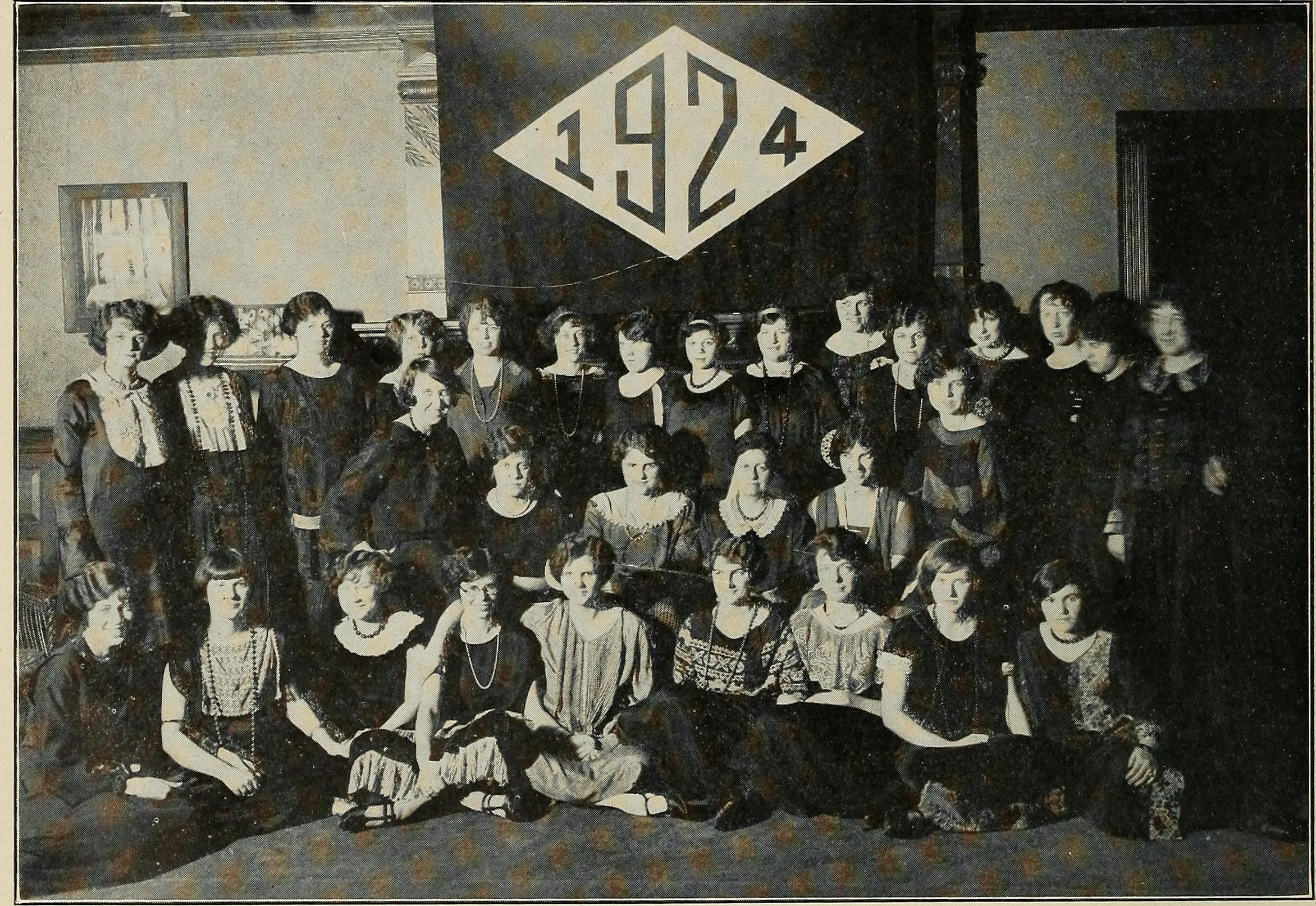This black and white photograph, dating back to 1924, captures an all-women graduating class meticulously arranged in a grand Victorian-era room. The backdrop features an eye-catching design—a diamond set on its side—showcasing the year "1924" prominently. Flanking this emblem are ornate marble columns which appear to frame a grand fireplace, adorned with draped fabric across its mantel.

In the foreground, the women are organized in neatly structured rows. The back row consists of women standing, while fewer women are seated in the middle row. The foremost row has women sitting on the ornate carpet, which is patterned with blue and red diamond shapes. These women are attired in quintessential 1920s flapper fashion, characterized by short, wavy or curled hairstyles and long, dangling necklaces that accentuate their period dresses.

Most of the women direct their gazes towards the camera, although a few are captured in candid angles. The room's lighter-colored walls add a soft contrast to the overall setting, with a prominent mirror visible to the left. The photo exudes a beautiful blend of period-specific elegance and academic accomplishment of the early 20th century.